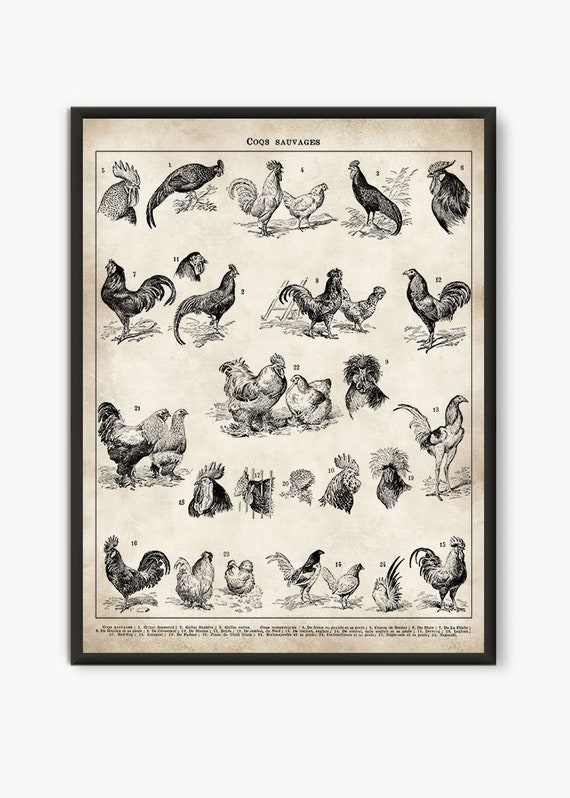The image depicts a vintage-style line drawing poster encased in a black frame, which might be made of either wood or metal. The top of the poster bears the caption "Coqs Sauvages," which is French for "wild roosters." The central part of the image is bordered by a square outline, containing over a dozen detailed black-and-white illustrations of various birds. These birds include roosters, chickens, and perhaps even peacocks, arranged in four to five rows. The illustrations show a mix of full birds and close-up views of their heads, with some profiles and others facing directly forward. The paper background appears to be yellowed and aged, adding to the vintage aesthetic. Additionally, there is a small text at the bottom of the poster, though it's not very legible.